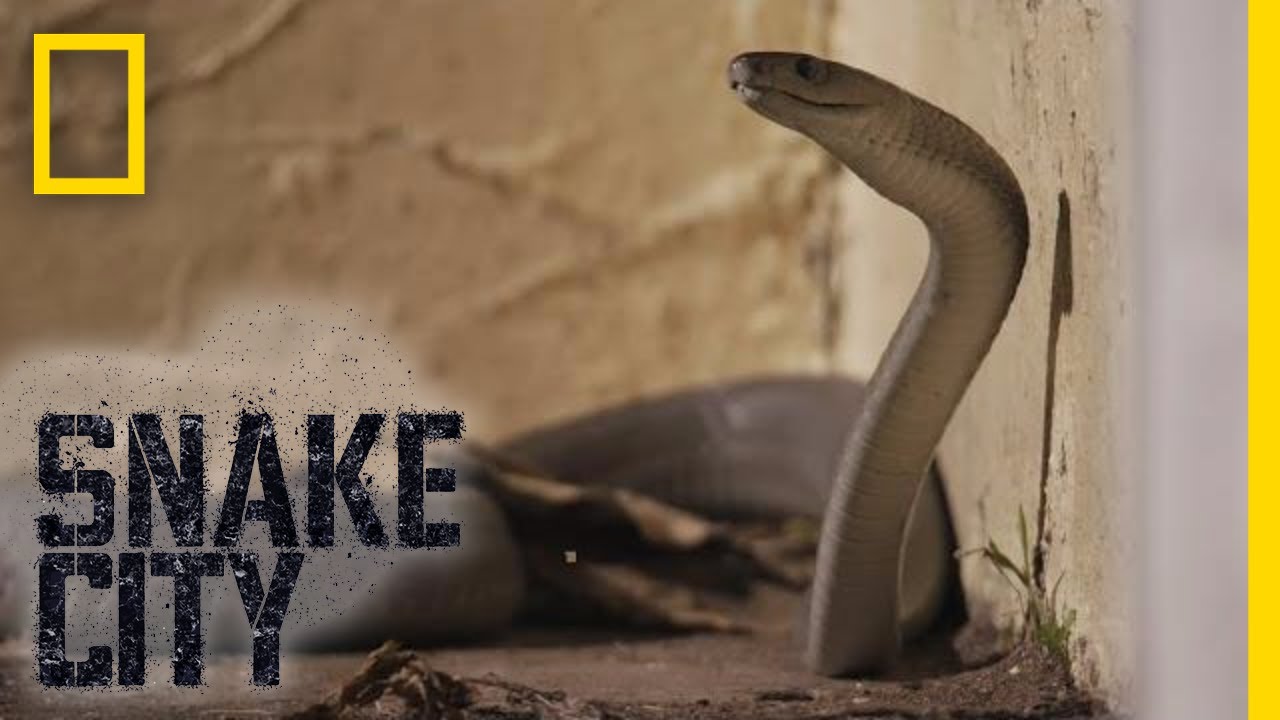The image is a vibrant, detailed color photograph most likely from National Geographic, as indicated by the signature long yellow rectangle in the top left corner and the large "Snake City" text in a black spray-paint stencil style in the bottom left corner. The focal point is a massive cobra stretched across the scene. Its head is lifted above the ground, facing to the left in profile, with an appearance almost reminiscent of a smile. The snake's body extends and coils against a textured, yellowish sandstone wall, indicating an outdoor setting on a dirt ground. The cobra, a white-brown hue, exudes an air of danger despite not showing its fangs or eyes prominently, implying its venomous nature. The photograph does not include any people, emphasizing the grandeur and solitude of the snake in its rugged environment.